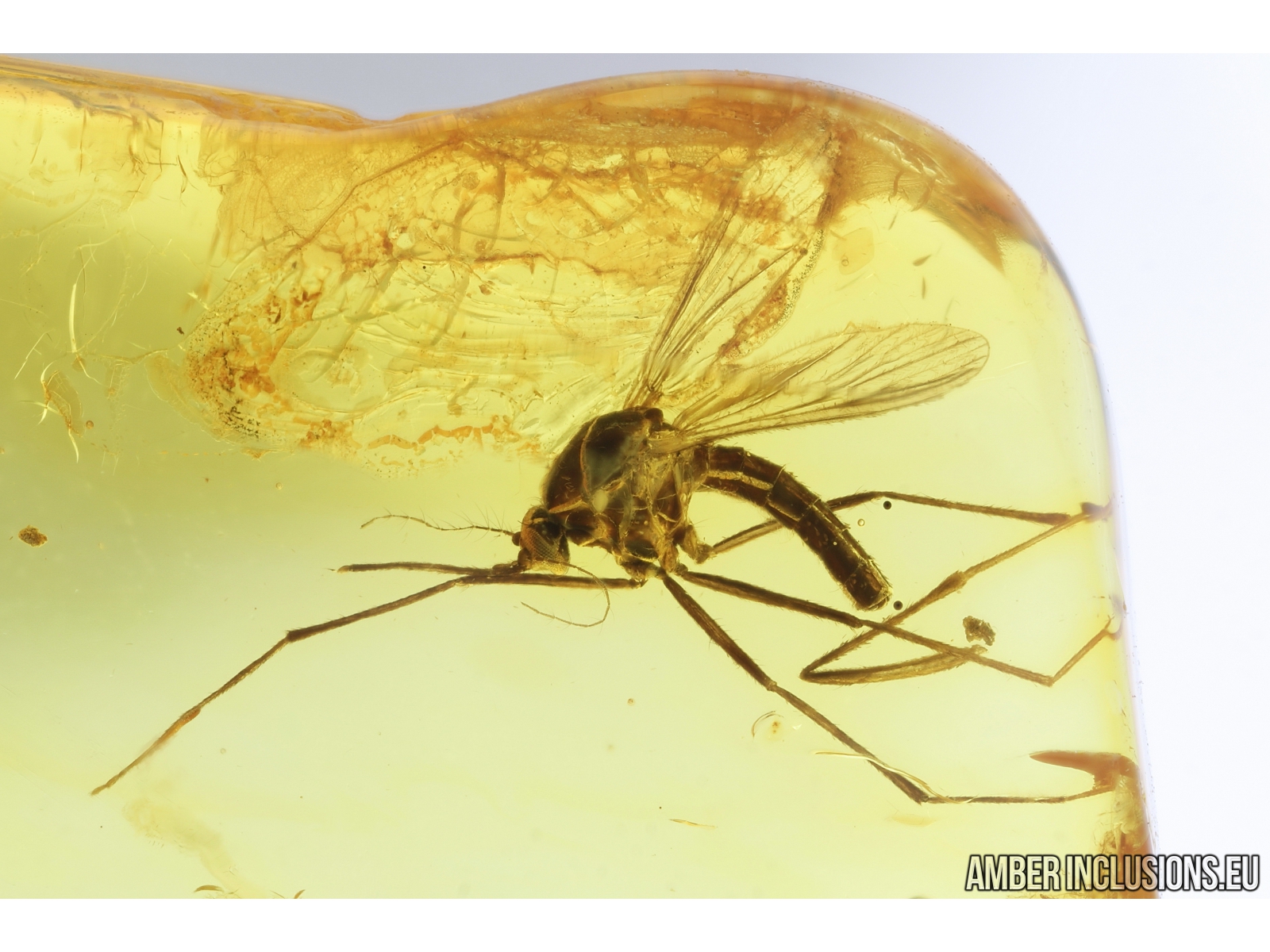This close-up image showcases a beautifully translucent piece of light yellow amber with darker yellow hues, encapsulating a fully-formed flying insect, potentially a mosquito. The insect, centrally located, maintains a remarkable level of detail, allowing viewers to clearly discern its body, wings, and legs. The image, notable for its high clarity, reveals not only the insect but also other inclusions and imperfections within the amber, contributing to its intricate beauty. The background is plain white, further emphasizing the subject. The bottom right corner features the text "amberinclusions.eu," indicating the source of the image.